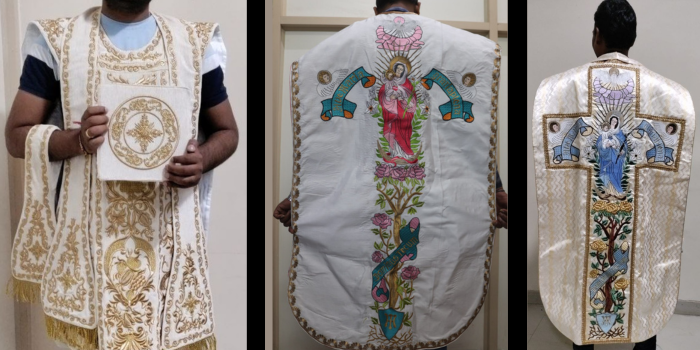The photograph presents three distinct portraits showcasing intricate religious garments, likely chasubles and stoles, set against a plain background. Each image features different designs, prominently displaying religious iconography.

On the left, there is an image of a man with brown skin, whose face is cropped out at the chin. He is dressed in layers including a black shirt, a light blue garment, and atop those a white drapery adorned with extensive gold embroidery. He holds a white square cloth embellished with a golden design. The garment he wears features a rich array of Christian symbols crafted with gold thread, demonstrating detailed hand embroidery, including a stole with gold accents.

The central image focuses on the back of another dark-skinned individual, showcasing a chasuble predominantly white with a golden border. The design, running vertically down the middle, features Jesus with a halo radiating golden rays, surrounded by floral patterns and greenery in hues of pink and blue. The composition includes additional symbols in gold, culminating in an emblematic representation of Christ.

On the right, the final photograph captures the backside of a man with black hair and skin, wearing another white chasuble. Central to this garment is a golden cross enclosing an image of Mary, encircled by blossoms and plant life painted in blues, yellows, and greens. The cross and its adornments cohesively merge to form the religious garment's centerpiece.

Collectively, these images emphasize the craftsmanship and religious significance embedded in the ceremonial garbs, reflecting their usage in Christian liturgical settings.